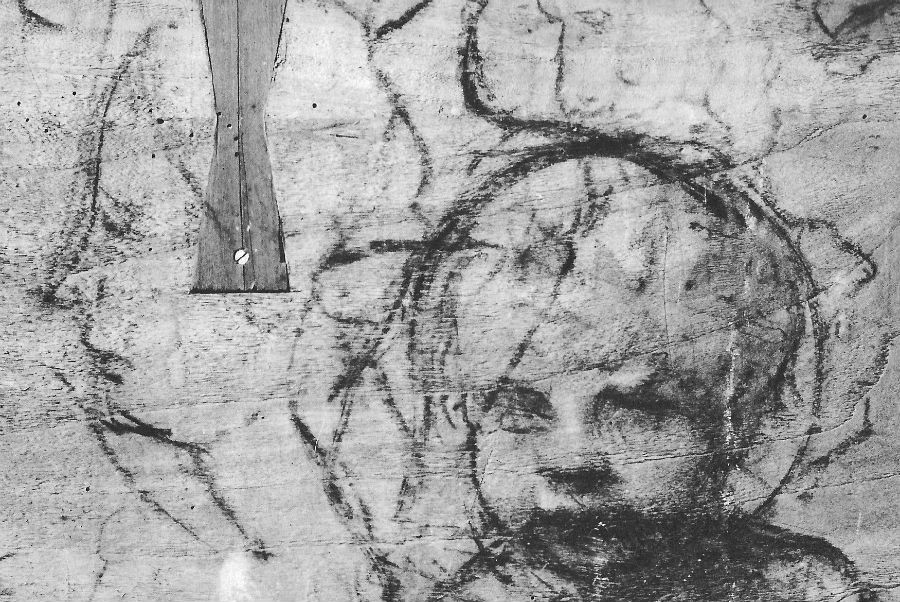This black and white image appears to be an intricate charcoal drawing or photograph on a gray wall. The artwork prominently features a well-detailed portrait of a young child, positioned on the bottom right. The child’s face is depicted in a somber, somewhat obscured manner, with only their head and a hint of shoulders visible. In the top left, there is a faint side profile of an adult's face, possibly female, rendered with a melancholy expression. The wall itself has a rough texture, adorned with random black, squiggly lines and other black markings. Additionally, there is a distinct wooden object, shaped like an hourglass, affixed to the wall with a screw on the left side, adding to the overall enigmatic and somber atmosphere of the image.